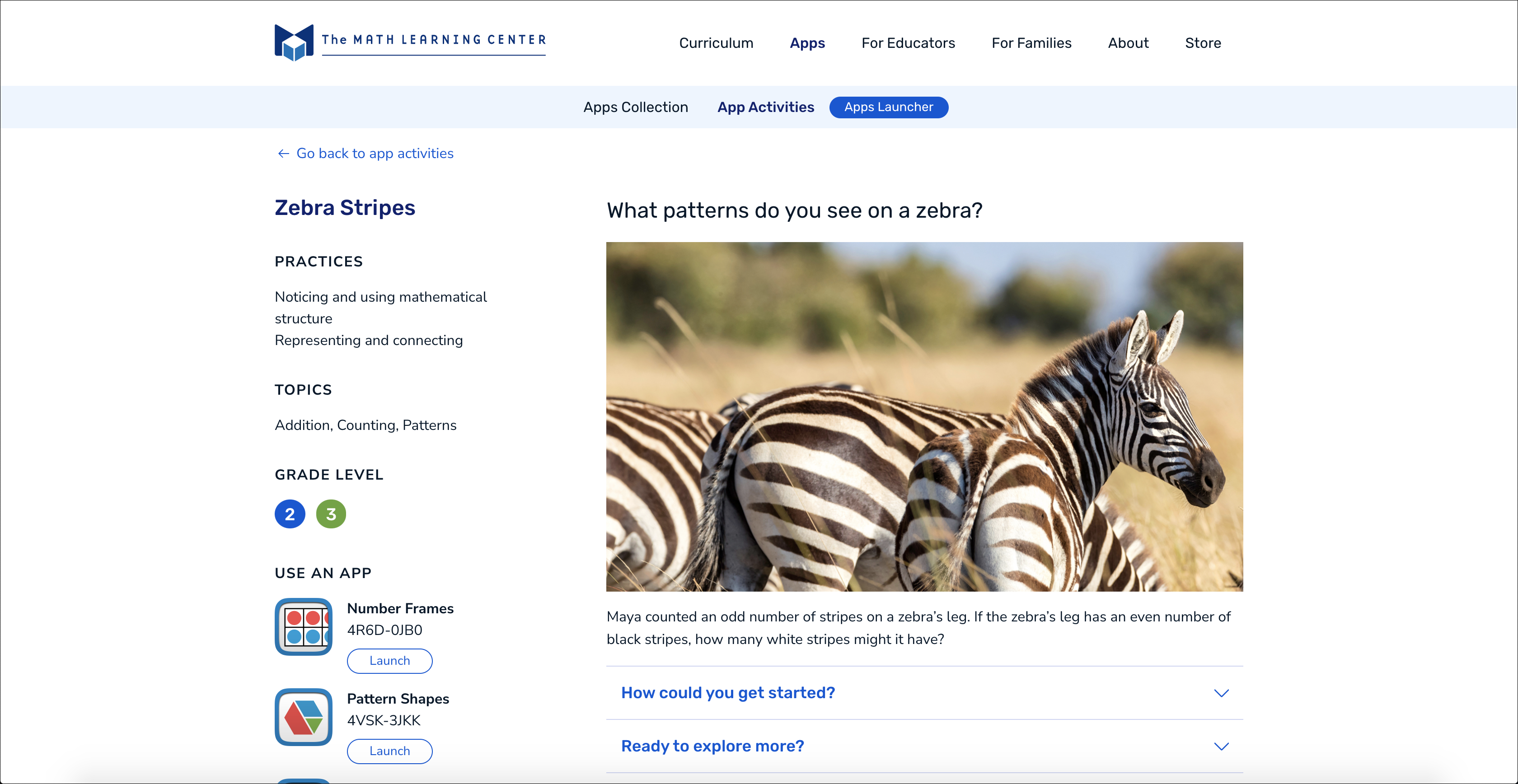This is a detailed screenshot of the Math Learning Center website, showcasing its layout and features. The page prominently displays the Math Learning Center logo, represented by a letter "M" accompanied by a small cube. The main navigation menu includes options for Curriculum, Apps for Educators, For Families, About, and Store. The "Apps for Educators" section is currently selected, revealing a sub-menu with options: Apps Collection, App Activities, and Apps Launcher. 

Highlighted is the Apps Launcher, depicted as a bright blue button. On the left side of the page, there's a detailed navigation menu with additional categories such as App Activities, Zebra Stripes, Practices, Topics, Grade Level, and Use an App. 

Within the Practices section, it lists Noticing and Using Mathematical Structure, Representing and Connecting Topics, Addition, Counting Patterns, and specific Grade Levels indicated by blue and green circles representing Grades 2 and 3. In the Use an App section, options include Number Frame and Pattern Shapes, accompanied by geometric icons and Launch Buttons.

To the right, the main content area displays a question prompt: "What Patterns Do You See on a Zebra?" This is accompanied by a photograph of zebras standing in a dry, grassy field. Below the image, a hypothetical scenario is presented: "My Account had an odd number of stripes on a zebra's leg. If the zebra's leg has an even number of stripes, how many white stripes might it have? How could you get started?" 

The prompt concludes with an invitation to explore more, followed by a series of dropdown arrows, which are blue text links, providing further options for exploration.